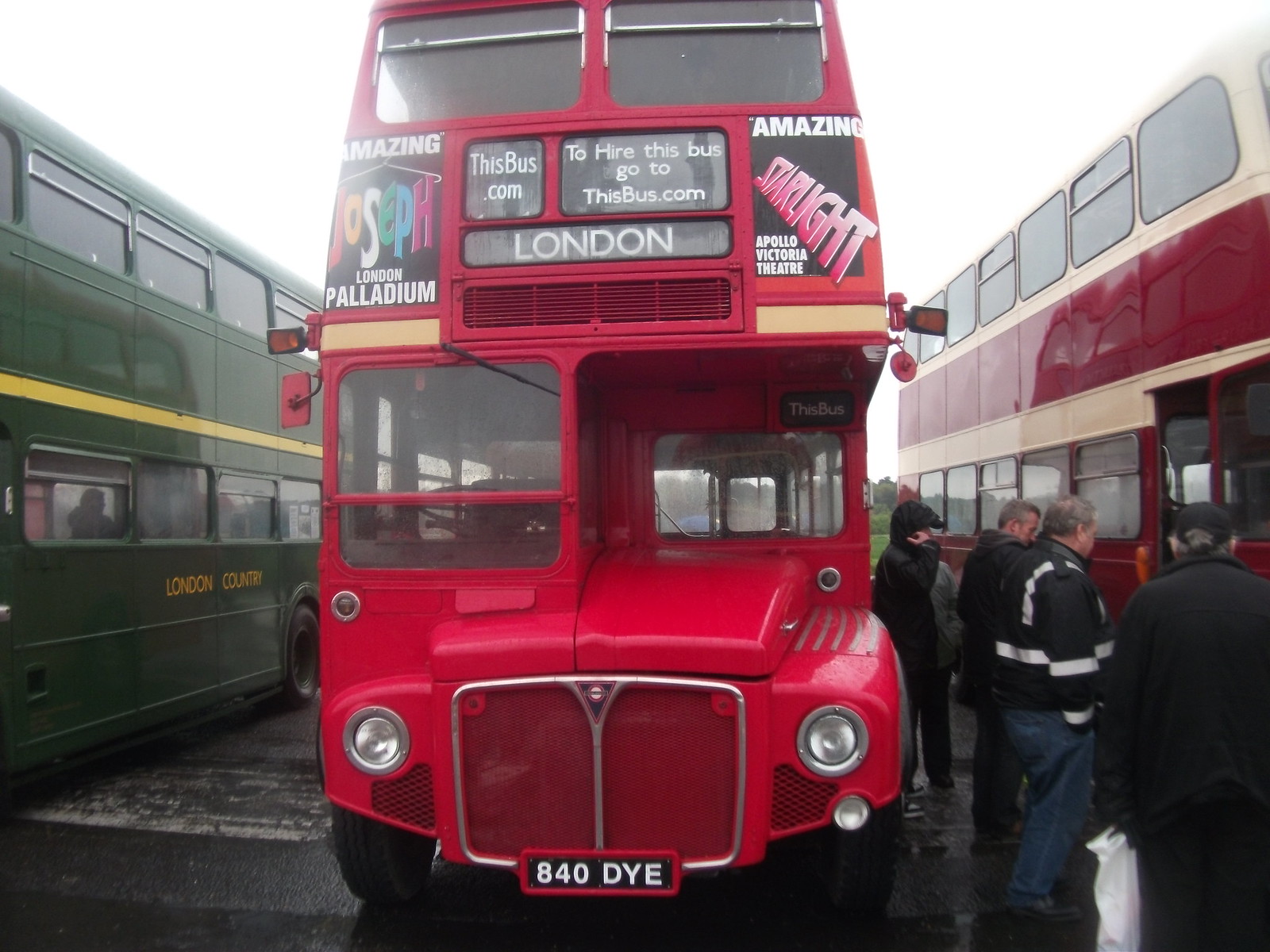The image features a vibrant red double-decker bus prominently displaying "London" and the number "845" on its front. Additional markings on the bus include "Starlight," "New Zealand," and "Palladium." To the bus's left, a green bus is visible, while a tan bus stands on the right. The tan bus, marked with "St. Lucie" and "bus.com," appears to be a newer model compared to the older, multi-colored bus beside it. Passengers are seen boarding this older bus on the right side of the image. The scene is set against a backdrop of a cloudy, overcast sky, adding a moody atmosphere to the bustling bus terminal.